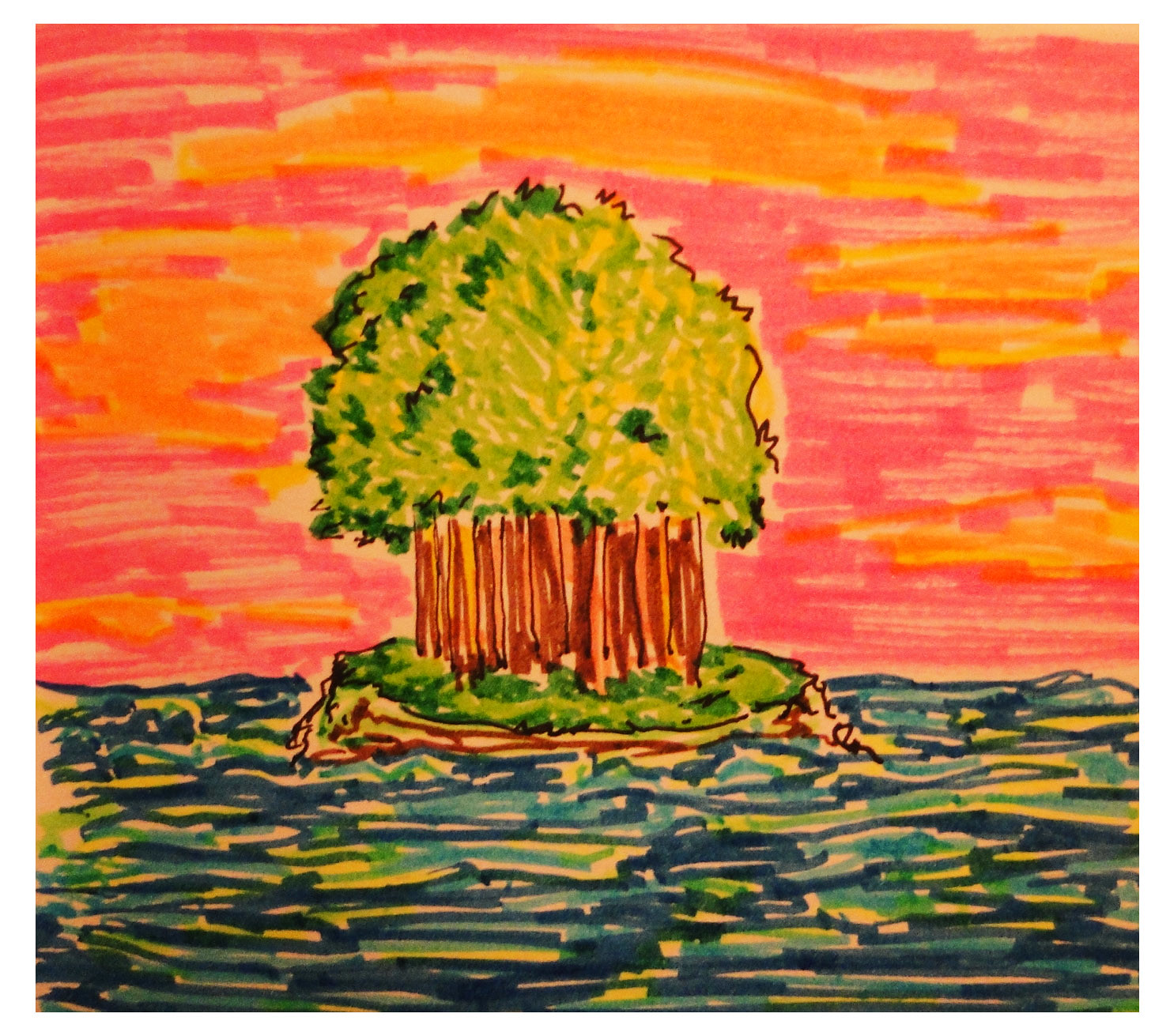The image depicts an intricately detailed drawing of a tree situated on a platform, which appears to be floating in the middle of a body of water. The lower portion of the drawing is predominantly colored in dark blue, with accents of light blue, green, and touches of yellow, creating a rippling water effect. Emerging from this aquatic base are hints of brown and light green lines, culminating in a circular green shape that serves as the surface of the platform. Rising majestically from this base are brown vertical lines that form the sturdy tree stump. The tree itself is adorned with foliage shaded in light green and yellow, capturing the dappled effect of sunlight filtering through the leaves. The background is a rich canvas of pink hues, interspersed with splashes of orange and yellow, adding a vibrant, almost ethereal quality to the scene.